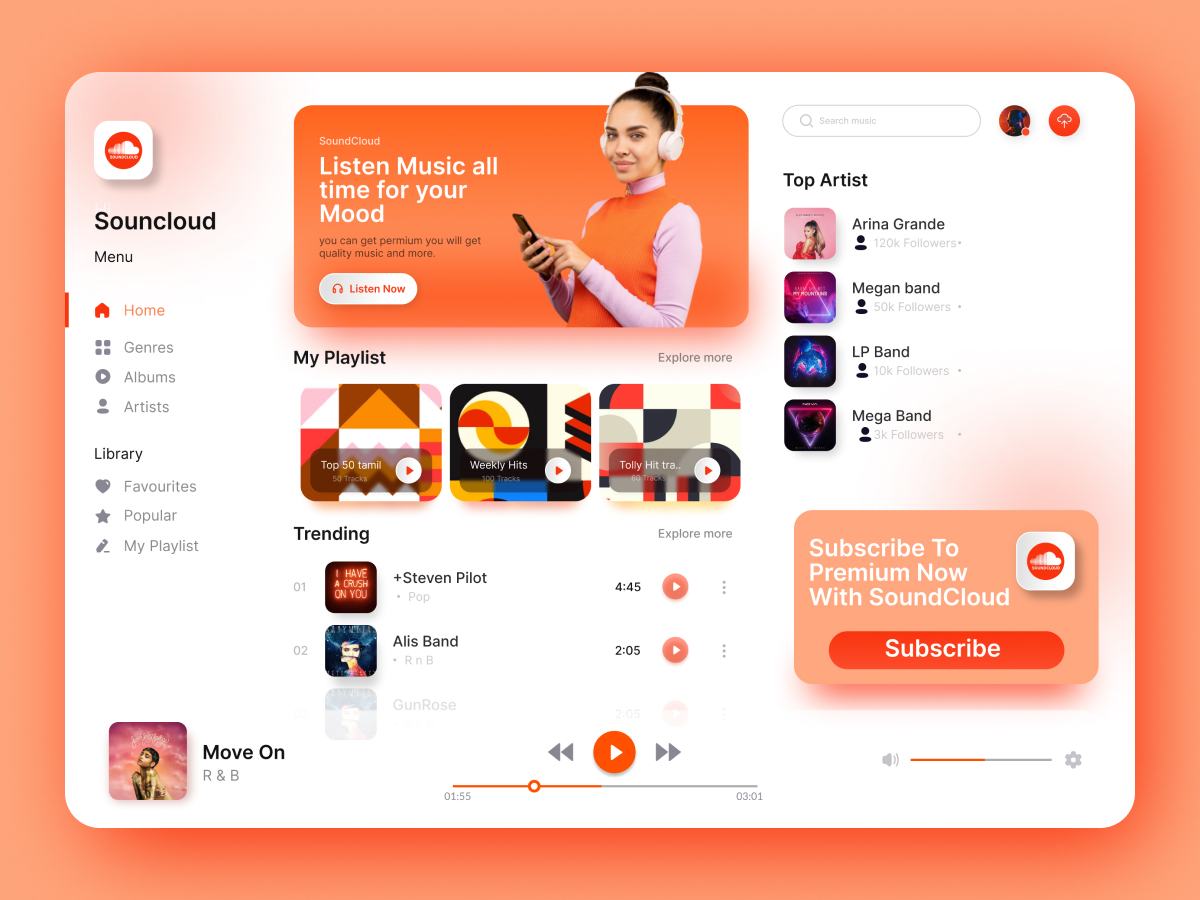The image showcases an updated layout of the SoundCloud interface. At the center, a prominent banner reads: "SoundCloud: Listen to music all the time for your mood." Below this tagline, there's an invitation to get premium, with a note promising "quality music and more." A white button labeled "Listen Now" is prominently displayed underneath the text. Adjacent to this, a section titled "My Playlist" features three different playlists, each visually distinct. Further down, a "Trending" section highlights a collection of popular songs and tracks, indicating current favorites among users.